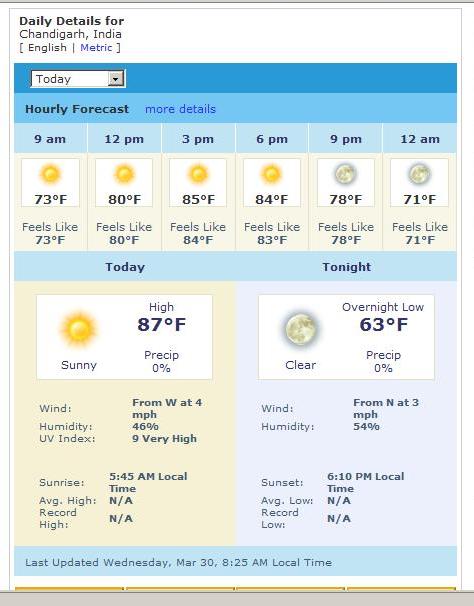Daily Weather Details for Changdor, India

In the top left corner of the image is the heading "Daily Details for Changdor, India." The forecast information is provided in English and metric units. Below this, additional weather details are categorized with black and blue text.

- **9 a.m.:** The temperature is 73°F, feeling like 73°F.
- **12 p.m.:** The temperature rises to 80°F under sunny conditions, feeling like 80°F.
- **6 p.m.:** It remains sunny, registering 80°F, though it oddly feels like 0°F.
- **8 p.m.:** Sunny with a temperature of 85°F, feeling like 80°F.
- **9 p.m.:** The temperature drops to 70°F under a moonlit sky.
- **12 a.m.:** Moonlit skies continue with a temperature of 71°F, feeling like 70°F.

For tonight, the forecast is sunny with a high of 80°F and a 0% chance of precipitation. The overnight low is predicted to be 6°F. 

- **Monday's Weather:** Clear skies are expected with no precipitation. The wind will come from the west at 4 mph, and the humidity level is 46%. The UV Index will be 10.5.
- **Additional Details:**
  - **Local Time Record at 9 a.m.:** The wind is coming from the north at 3 mph with a humidity level of 54%. 
  - **Sunset:** Recorded locally at 6 a.m. 
  - **Last Updated:** Wednesday, March 30th at 8:25 a.m. local time.

The image also features a color theme: a brownish-red hue on the left side transitioning to blue on the right side, with a gray bar at the bottom of the image.